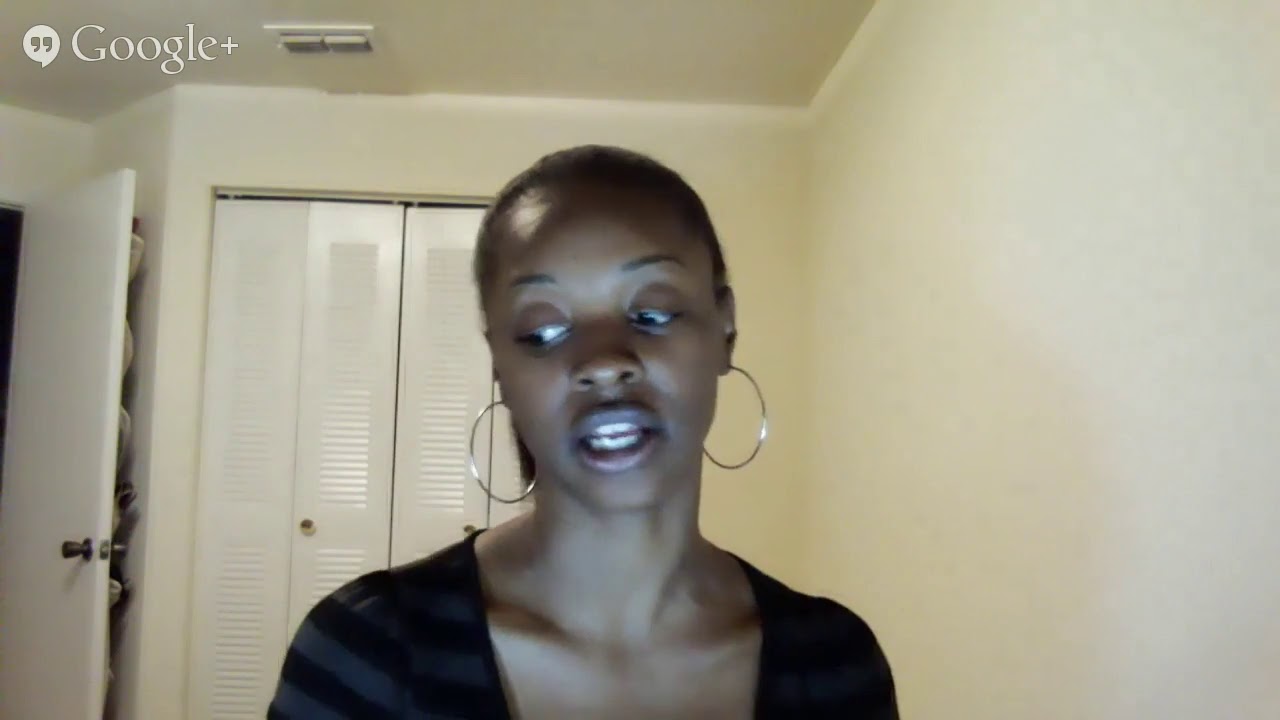This image is a wide rectangular screenshot of a Google Hangouts video chat, featuring a woman of African American descent in a room with beige-yellowish walls. The image captures her head, shoulders, and upper chest as she looks towards the bottom left corner. She has short black hair, is wearing prominent gold hoop earrings, and is dressed in a black shirt. Her face is somewhat illuminated by the computer screen she’s looking at. 

In the background, there is a white closet with four narrow vertical rectangular panels with shutters, each equipped with a golden doorknob. To the left of the closet, there is a white door which appears to be the entrance to the room. Beige walls and a light-colored ceiling frame the scene. On the left side of the image, near the top, the words "Google+" are visible, accompanied by a quotation mark-like symbol, emphasizing the Google Hangouts interface. The room appears fairly empty, with distinct creases on the walls and ceiling visible, creating a simple yet detailed backdrop for the video call.